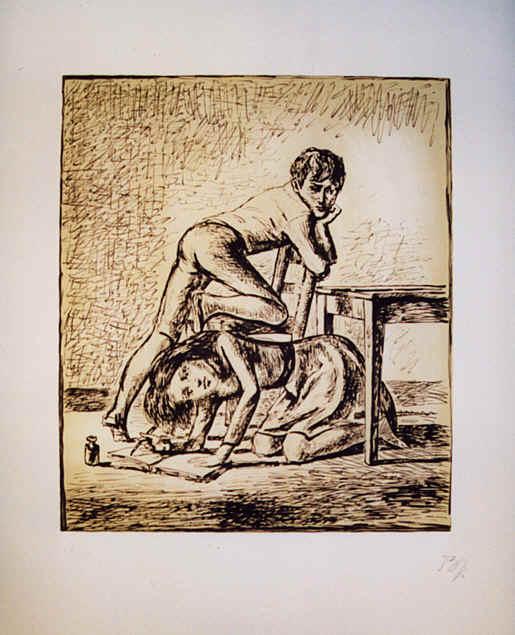The image is a detailed sketch, possibly created with pencil, black ink, or charcoal, on brownish-tan colored paper. It features two children, a little boy and a little girl who are seemingly young teenagers. The scene is set against a plain wall and floor, void of other significant items, creating a minimalist background.

The girl is positioned on the floor, her legs and bottom partially under a desk or table, while the upper part of her body extends outward. She is on her hands and knees, examining a book placed on the floor in front of her. In her right hand, she holds a quill or ink pen, and an ink jar is also visible nearby. She is dressed in a long-sleeved dress that is cinched at the waist, and she looks to the side, deeply engrossed in her activity.

The boy, dressed in capri pants and a shirt, is leaning over a chair situated behind the girl. His right knee is bent and resting on the chair while his left leg stretches out on the floor. He has his right arm wrapped around the back of the chair, and his head is nestled in his left arm, with a contemplative expression as he looks down at the girl. 

The sketch is characterized by bold outlines and extensive use of line shading, conveying a dynamic and somewhat chaotic energy through its etching style.